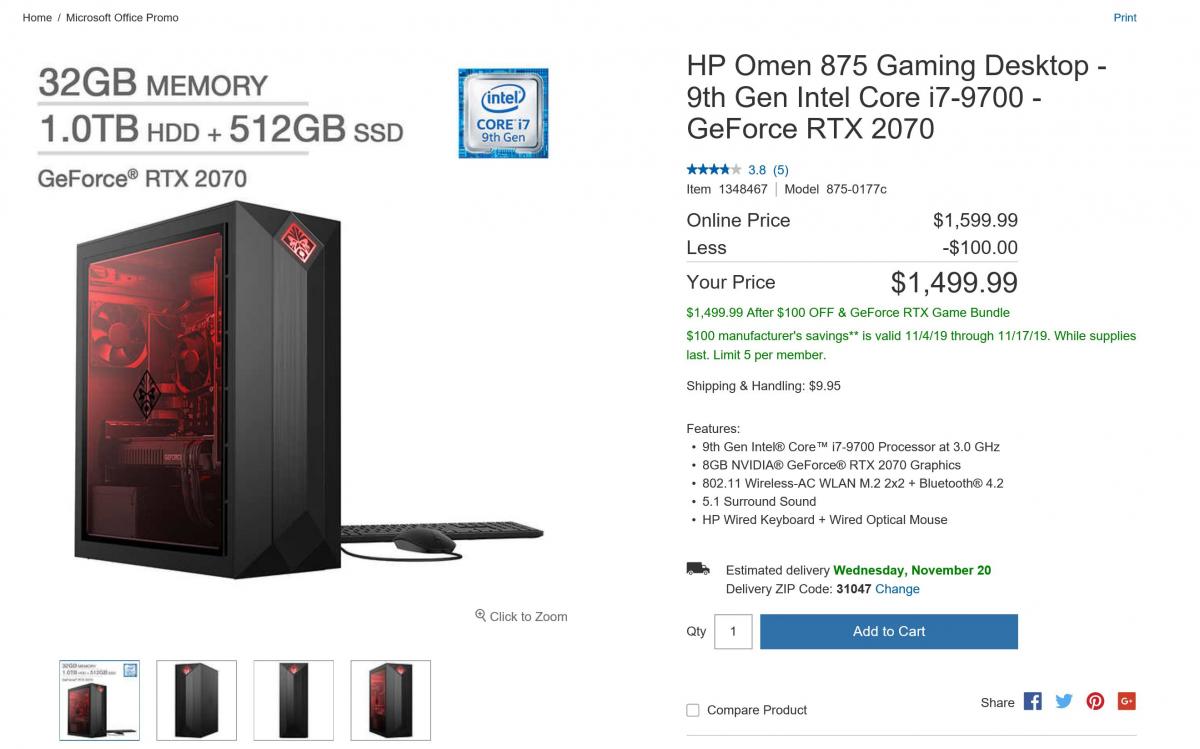The image depicts an advertisement for an electronic product, specifically a gaming desktop. The majority of the picture features a white background. At the top of the ad, there is fine black print that reads "Home / Microsoft Office Promo." Just below, in larger black letters, it states "32 GB (gigabyte) memory." A gray line separates this from the subsequent text, which lists "1.0 TB HDD + 512 GB SSD." Further down, it mentions "GeForce RTX 2070."

The central part of the image showcases the internal components of the computer, including the CPU (central processing unit). To the side of the CPU, a mouse is visible, along with a thin keyboard. Below this section, there are four small images, presumably clickable, that offer different views of the product.

The product being advertised is the "HP Omen 875 Gaming Desktop" featuring a 9th Gen Intel Core i7-9700 processor and a GeForce RTX 2070 graphics card.